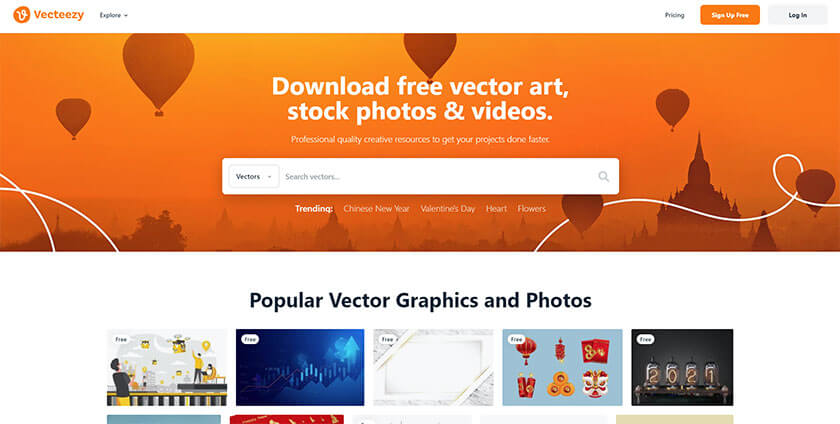The screenshot captures a section of the Vecteezy website, prominently displayed on a computer screen. In the upper left corner, there is the Vecteezy logo followed by a dropdown menu labeled "Explore". On the right side of the menu bar, there are three clickable buttons: "Pricing," "Sign Up Free," and "Login." Dominating the center of the screen is an inviting orange background adorned with festive balloons and an illustration reminiscent of a Disney World castle. Overlaying this background is bold text that reads: "Download Free Vector Art, Stock Photos, and Videos – Professional Quality Creative Resources to Get Your Projects Done Faster."

Beneath this text lies a white search box with an option to search for vectors. This search box includes a dropdown menu, suggesting that users can search for other types of media as well. Below the search bar, a trending section features popular search terms such as "Chinese New Year," "Valentine's Day," "Heart," and "Flowers." 

Further down, there is a heading labeled "Popular Vector Graphics and Photos," under which a selection of five images is visible, with the beginnings of a second row peeking into the frame. The user interface evokes a user-friendly and visually appealing platform designed to help users quickly find high-quality creative resources.